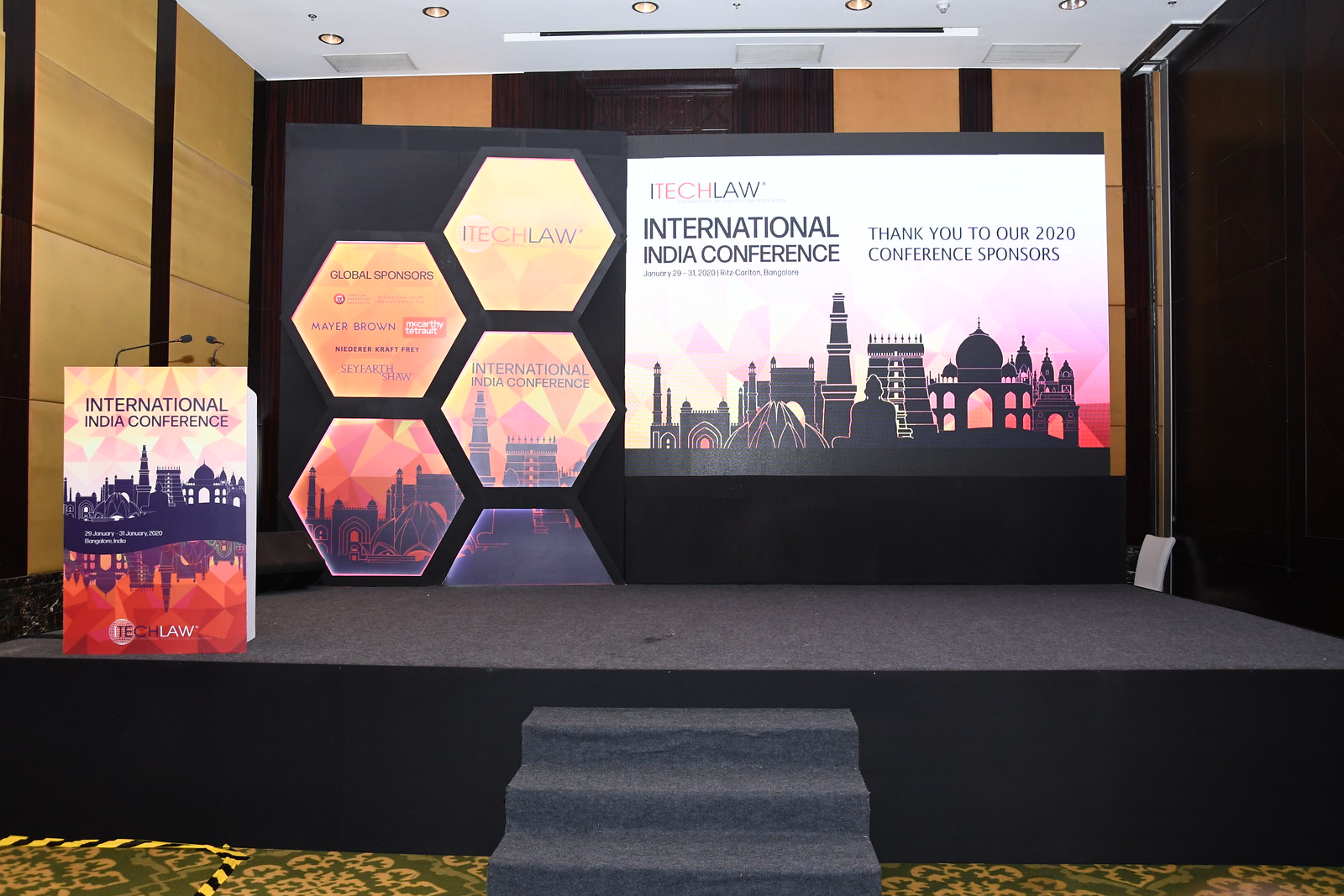The stage, which is black, has three black steps leading up to it. The backdrop is predominantly black, featuring five gold octagons on the left half. Within these octagons are words and images, some depicting cityscapes. On the right half of the backdrop, there is a horizontal poster that reads "I-Tech Law International India Conference" with a message thanking the 2020 conference sponsors. This poster also includes a picture showcasing buildings of Indian architecture. A podium is located at the lower left corner of the stage, adorned with the same architectural imagery and the inscription "International India Conference." The backdrop also features some wooden elements, adding a contrasting texture to the predominantly black scenery.